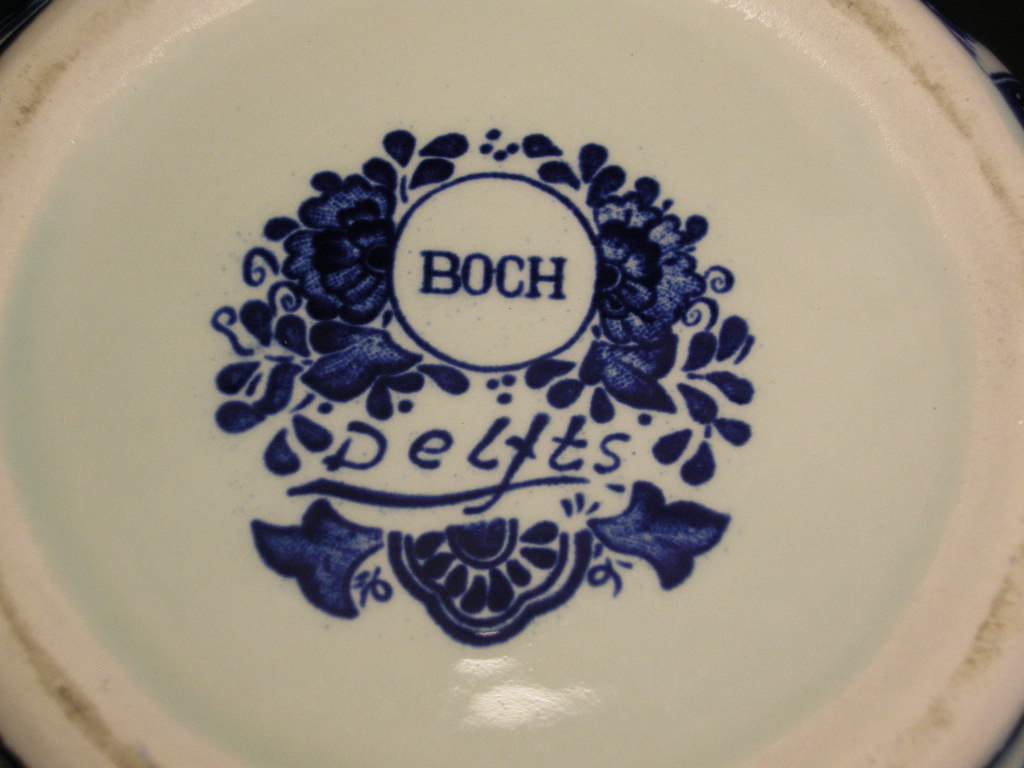The photograph features a rectangular image, approximately four or five inches tall by six inches wide, showcasing the bottom of a piece of ceramic dishware. The dishware appears to be white and rounded, though the full shape—whether it is circular or oval—is partially cut off at the sides, top, and bottom. The rounded edges are slightly visible along with a bit of the outside, suggesting it might be a bowl or a plate. Around the rim of the dishware, there are noticeable darkened spots, indicating where it has been worn from frequent contact with surfaces.

In the center of the dishware is a notable blue design that appears to be ornate and floral, incorporating flowers and leaves. This design surrounds a white circle with a blue border. Inside this white circle, the blue text reads "BOCH." Below this circle, there is additional text that reads "D-E-L-F-T," appearing to incorporate a stylized "J" or "T" which is crossed and underlined. Beneath this text, there are more blue leaf designs.

Overall, the blue central design is intricate and forms an imperfect circular shape. While the rest of the dishware remains white, the edges show signs of dirt and aging, suggesting that the item has been used frequently over a period of time. The piece combines both a utilitarian function and an aesthetic appeal with its central floral motif and historical inscriptions.